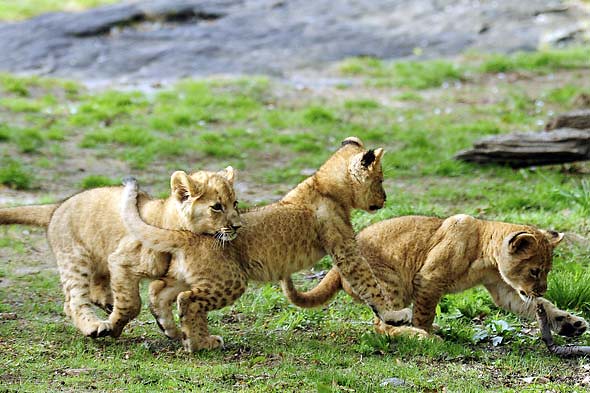The photograph captures a dynamic close-up of three playful wildcat cubs, all fuzzy tan with little black spots, suggesting they are either lions, tigers, or cheetahs. These energetic cubs are positioned in a grassy outdoor setting, dotted with sparse patches of bare ground and framed by gray, rocky outcrops in the background. The central focus of the image reveals one cub having an intense nose-to-nose encounter with a small snake that has its neck and mouth raised, staring back at the cub. This cub seems to be receiving a warning from the middle cub, who has his face resting on the back of the first cub. The middle cub's tail is intriguingly wrapped around the neck and back of the first cub, indicating a collision or playful pounce. The third cub, on the far right, is captured in a state of curiosity, crouching with his paw extended and his eyes fixed on the snake, as if anticipating what will happen next. The scene exudes a sense of playful tension and curiosity, underscored by the idyllic outdoor backdrop of grass and rocks.